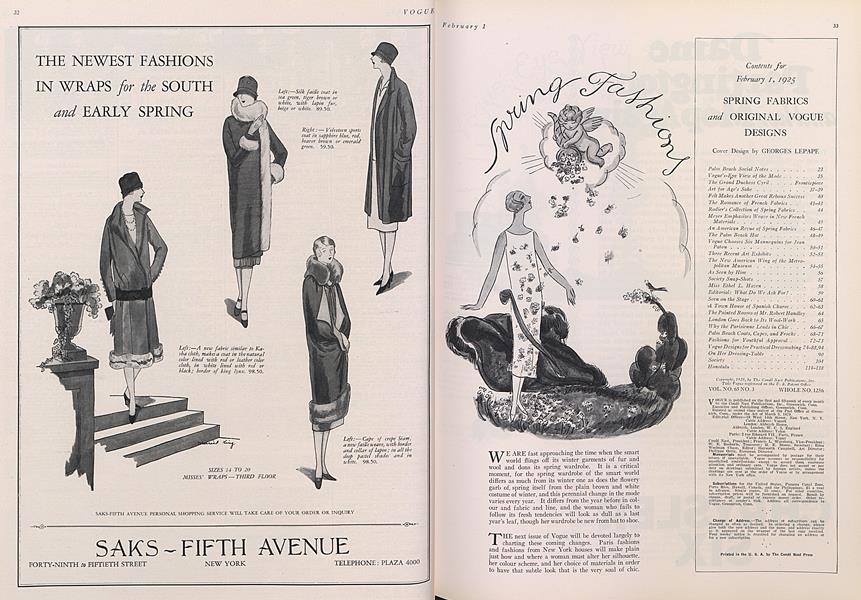This black-and-white image appears to be a vintage advertisement from a 1930s-1950s Vogue magazine, featuring a two-page spread promoting the latest fashions from Saks Fifth Avenue. The left page is outlined in black and titled "Newest Fashions and Wraps for the South and Early Spring." It showcases several women modeling stylish jackets, trench coats, big scarves, and heels, with some of them elegantly descending stairs adjacent to a post adorned with flowers. Detailed captions and descriptions in black ink are placed next to each model, providing further insight into the outfits.

On the right page, the focus shifts to spring fashions. At the top, ornate script text forms a semicircle around a charming Cupid, who is depicted showering a woman in a long white dress with flowers from above. This woman stands in a grassy area, accompanied by additional whimsical elements such as a bird perched on a flower and what appears to be a snake wrapped around her. Beneath this illustration, there is an article about "Spring Fabrics and Original Vogue Designs," offering detailed information and prices for the various fashion items advertised.